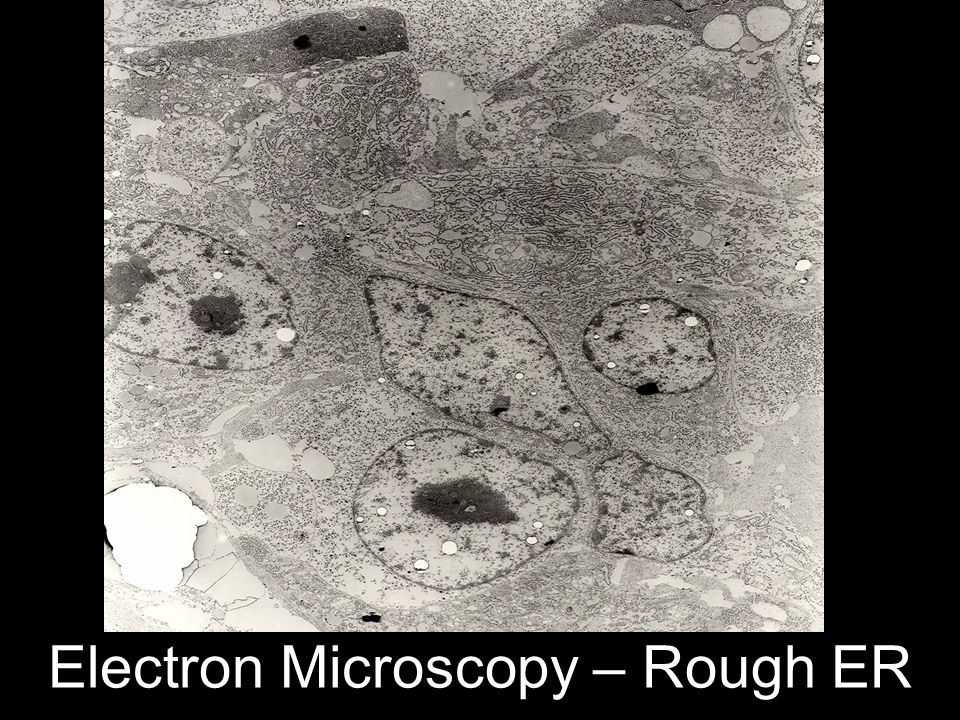The image showcases a highly magnified, black-and-white electron microscopy scan, likely of biological cells, specifically focusing on the rough endoplasmic reticulum (ER). The background is solid black, providing a stark contrast to the grayscale cellular imagery positioned prominently at the center or top of the screen. The cells exhibit a variety of shapes, including circular, oval, and one resembling a diamond shape amongst more detailed striated structures. These intricate formations, though difficult to discern clearly, suggest a micro-level examination of cellular components. Large white text at the bottom reads "Electron Microscopy - Rough ER," indicating the nature of the scan. The overall presentation, complete with a black border framing the scene, suggests an educational or medical presentation slide aimed at highlighting these microscopic details.